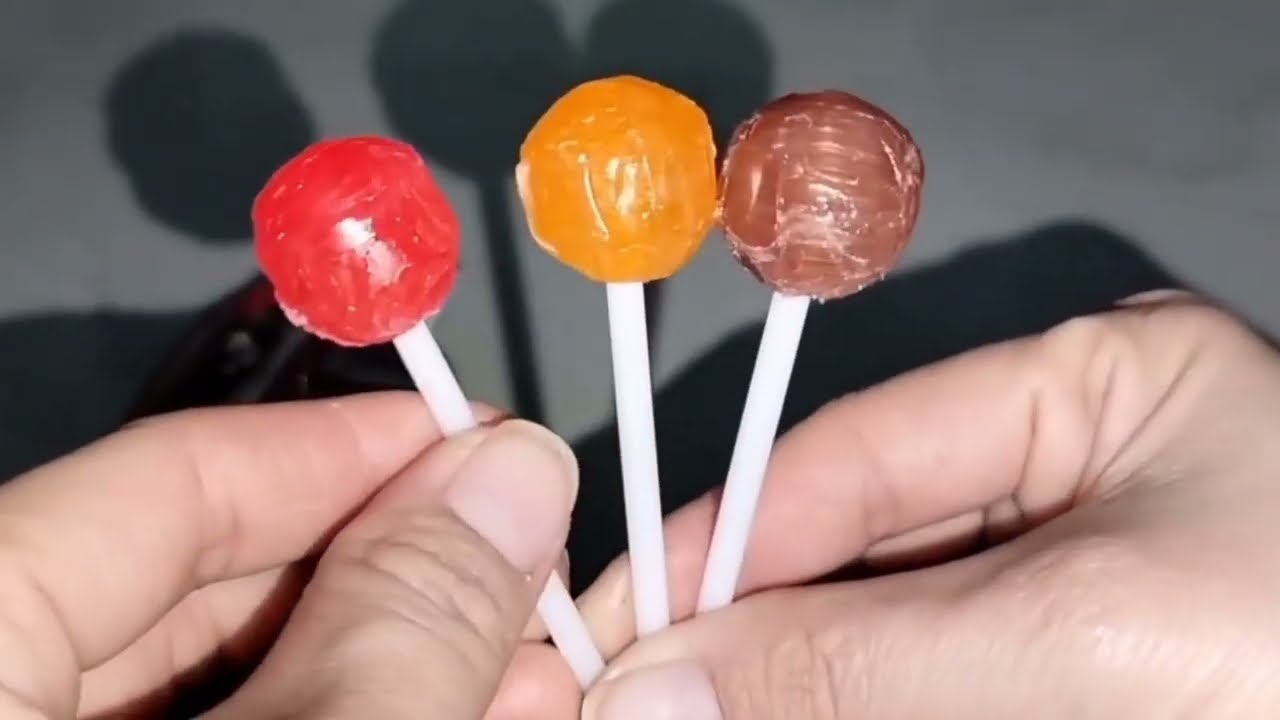In this detailed indoor photograph with a gray-painted wall as the background, the focal point is a pair of hands, which appear to be male and of Caucasian descent, holding three Tootsie Roll-type lollipops with long white fingernails. The hands, illuminated by a camera flash or similar lighting from behind the camera, cast shadows on the wall. The left hand pinches a red lollipop between the thumb and forefinger. The right hand grips both an orange lollipop, likely butterscotch, and a brown lollipop, possibly root beer-flavored, with its thumb and forefinger. The shadows of the hands and lollipops are clearly visible against the gray background, adding depth to the image. The precise positioning suggests the red lollipop might be slightly pulled away from the other two, emphasizing the individual colors and flavors of each candy.